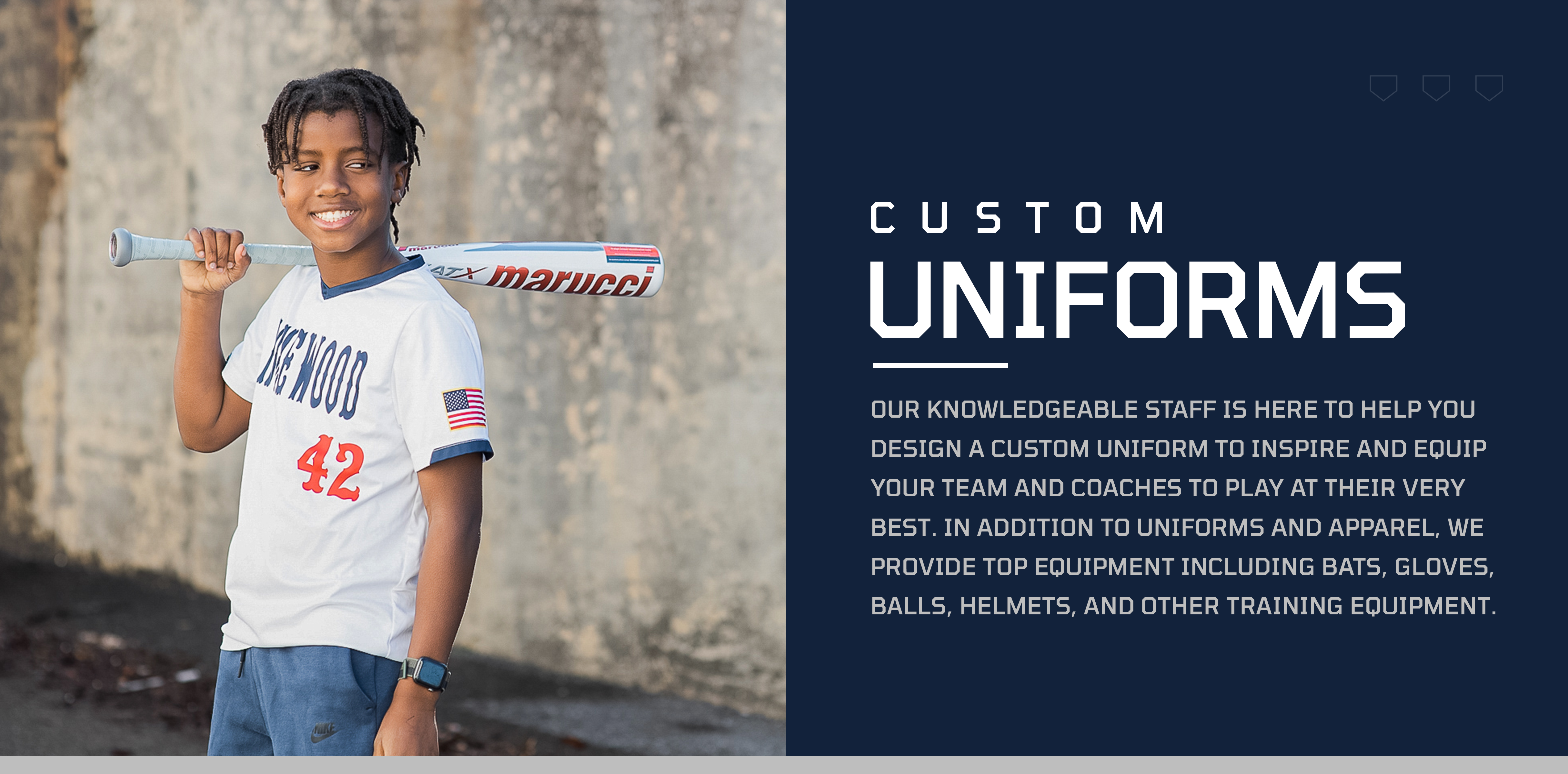The image is a rectangular ad for custom sports uniforms, divided into two distinct sections. On the left side, a photograph depicts a young black boy, estimated to be around 14-15 years old, smiling brightly as he holds a white Marucci baseball bat balanced on his right shoulder. He is wearing a white short-sleeved baseball shirt adorned with the number 42 in red and dark blue lettering above it, along with an American flag patch on his left sleeve. Completing his attire, he wears jeans and a watch on his left wrist. The backdrop behind him is a modeled gray wall, and he is facing left while looking to the right. On the right side of the image, against a very dark blue background, white text prominently reads "Custom Uniforms." Beneath this, additional smaller white text provides details about the services offered: "Our knowledgeable staff is here to help you design a custom uniform to inspire and equip your team and coaches to play at their very best. In addition to uniforms and apparel, we provide top equipment including bats, gloves, balls, helmets, and other training equipment." The ad is designed as a postcard-sized promotional material.